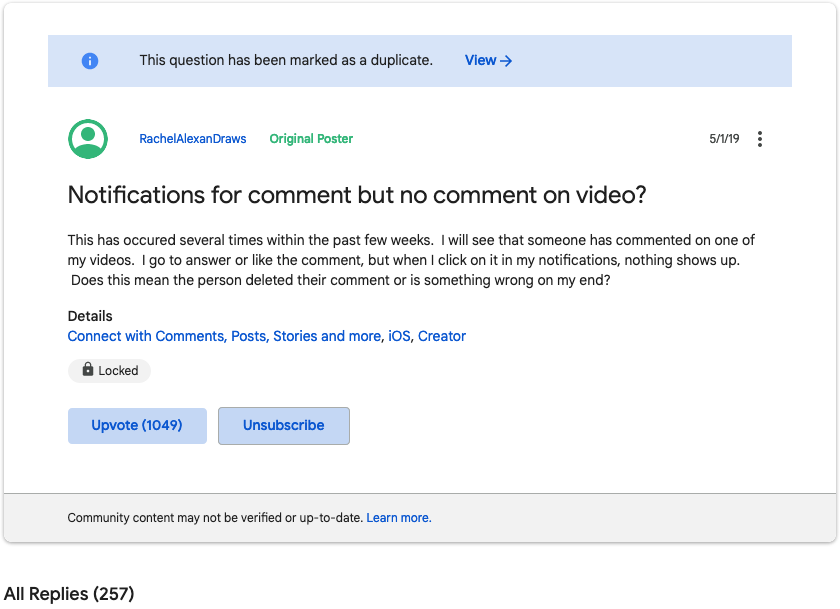The image features a predominantly white background with a bold blue header. Within the header, there is a white eye icon encircled by a blue ring. The text prominently reads, "This question has been marked as a duplicate." Below this, a blue text link titled "View" and a blue right arrow icon are visible. 

Further down, the phrase "Rachel Alexandra's original poster" is displayed in green, alongside a date stamp of "5/1/19". Three vertical dots can be seen, suggesting additional options. There is a notification icon indicating a comment that hasn't been responded to, with no actual comment displayed on the video.

The lower portion of the image indicates that similar instances have occurred multiple times recently. The person mentions receiving notifications about comments on their videos, but upon attempting to view them through the notifications, no comments appear. The user questions whether this could mean the comment was deleted by the poster or if it might be an issue on their end.

Additional details are provided in a series of blue-highlighted words: "connect with comments, post stories, and more, iOS," as well as "creator." The image also displays a grey oval shape, which appears to be a button and an image of a lot.

At the bottom of the image, there are two blue rectangles — one labeled "Update (1049)" and the other labeled "Subscribe."

This caption provides thorough and vivid details of the components and layout of the image described.